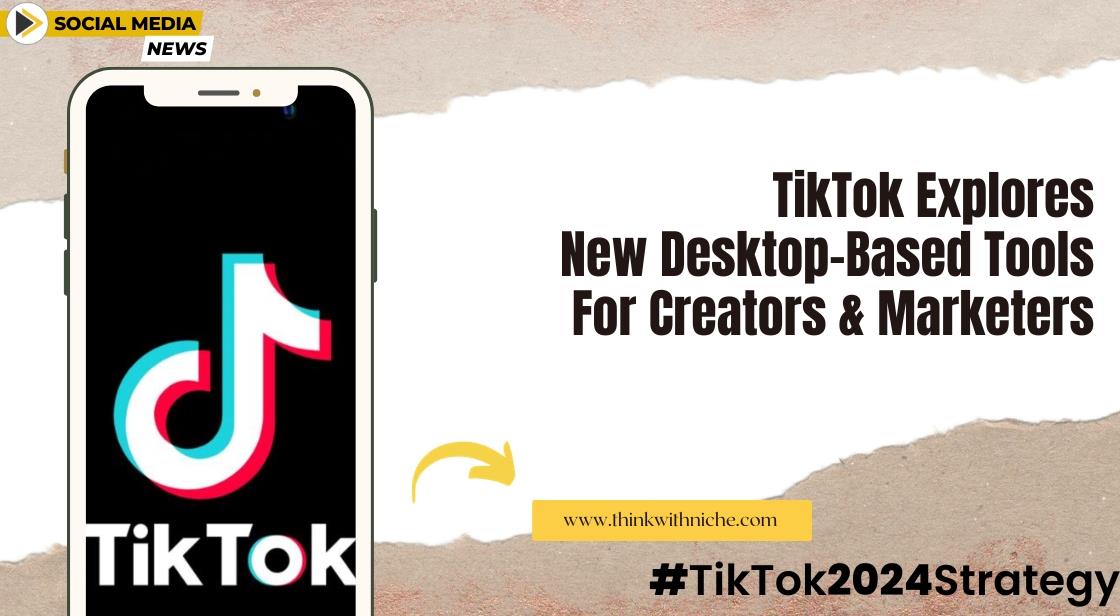The image features a predominantly beige box with a varied color scheme. The top and bottom sections are beige, while the middle section is of a slightly darker beige. In the upper left-hand corner, the phrase "Social Media News" is displayed in black font. To the left, there is an outline of a phone with a white body, black border, and black screen, featuring the word "TikTok" in the middle. Below the phone image, in bold black letters on a white background, the text reads: "TikTok Explores New Desktop-Based Tools for Creators and Marketers".

Further down, a yellow arrow points towards a yellow rectangle. Inside the yellow rectangle, the URL "www.thinkwithniche.com" is displayed in black font. The bottom part of the box returns to a darker beige hue. Here, a black hashtag symbol (#) is followed by the text "TikTok 2024 Strategy", with a capital "T" for TikTok and a capital "S" for Strategy, all in bold black font.